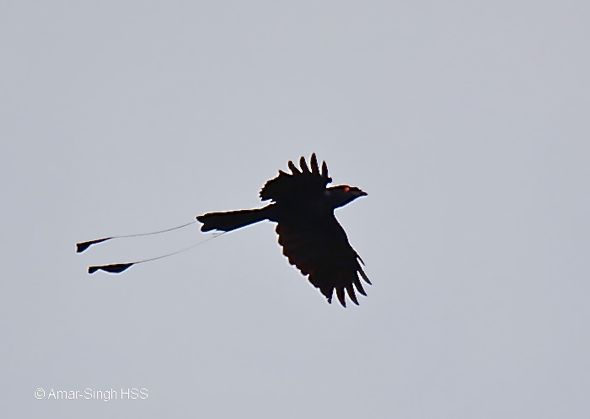This is a photo of a bird in mid-flight with its wings ruffled out against a bluish-purple, overcast sky. The bird, resembling a black crow with an intense red eye, flies from left to right. Its long tail and even longer ribbon-like extensions trail behind, mimicking the tails of a kite. The image is dark, making it difficult to discern fine details beyond the bird's predominantly black coloration. The composition exudes a solitary aura with only the bird in view. In the bottom left-hand corner, a faint white text reads "Copyright Amar Singh HSS."